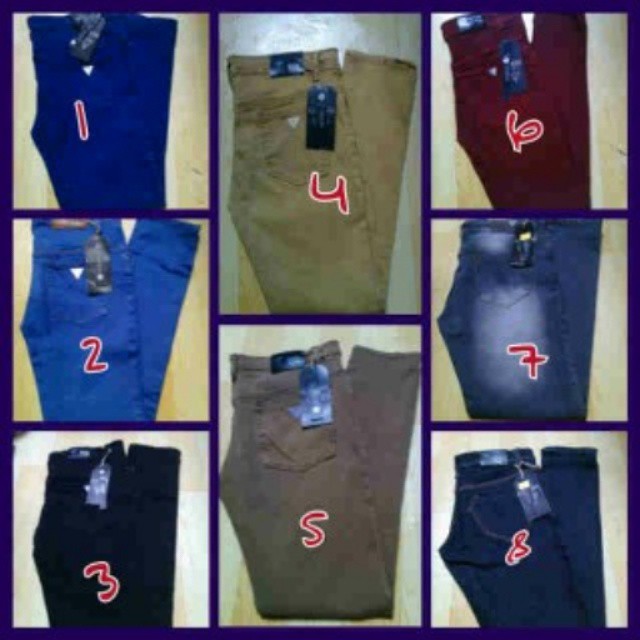The image is a square, sectioned into eight smaller, realistic photographs of folded pants, each labeled with red numbers from one to eight. The layout consists of three columns: the left and right columns each contain three vertically stacked rectangles, while the middle column features two larger vertical rectangles. The pants vary in color: Number one is navy blue, two is cornflower blue, three is black, four is tan khaki, five is gray-brown, six is crimson, seven is standard denim, and eight is dark indigo denim. Notably, the tan khaki and gray-brown pants in the middle column are the largest images, emphasizing their central position in this visually cohesive collage. The image has a blue border, adding structure to the presentation.